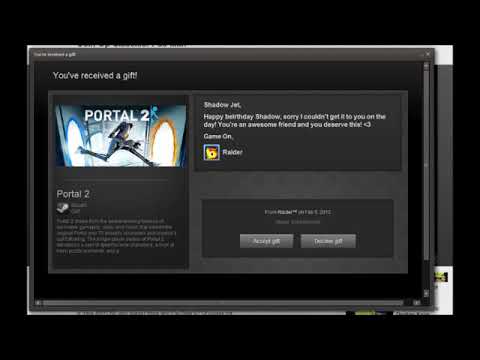The image is a low-resolution screenshot from the Steam platform showcasing a birthday gift message. The background is predominantly black, with a central gray and black rectangular interface indicative of Steam's dark mode. At the top left of this interface, there's a blue-toned image of a person running through archways, with "Portal 2" written above it. Beneath the image, a message is partially visible, though blurry: "You've received a gift. Happy birthday, Shadowjet! Sorry I couldn't get it to you on the day. You're an awesome friend and you deserve this." The message is adorned with a small heart symbol. Below the text, there are two gray buttons with white text, labeled "Accept Gift" and "Decline Gift". On the right side, there is an orange-colored patch, although its details are unclear. The overall color scheme includes black, white, gray, blue, yellow, and orange.